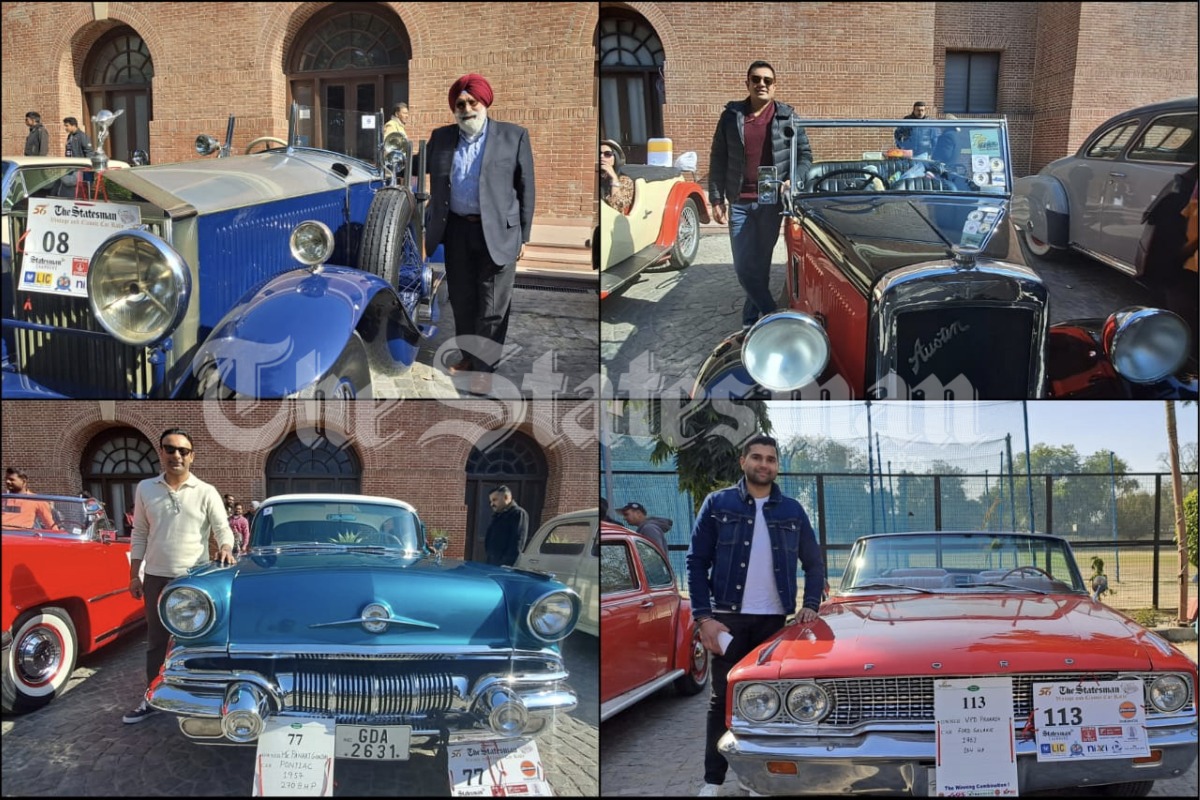This image, titled "The Statesman" as indicated by the watermark across the middle, appears to depict a car fair with four classic cars and their respective owners positioned in front of various backgrounds. Each section of the photograph showcases a different man with his car:

- The top left panel features a dark blue car from the 1920s, parked in front of a brick building with arched windows. An elderly gentleman, adorned in a grey suit, grey pants, red turban, white beard, and sunglasses, is standing proudly beside it.
  
- The top right panel shows a black and red Aston Martin sports car, identifiable by its two front lights and right-hand driver's side. The car enthusiast next to it is a man in his 40s, dressed in a black jacket, dark red sweater, and jeans. This car is numbered 8.

- The bottom left panel displays a metallic blue car from the 1950s or 1960s with a white top, standing in front of a similar brick backdrop. The man beside this car is wearing sunglasses, a white shirt, and black pants.

- The bottom right panel captures a red convertible from the 1970s in front of what might be cricket nets or athletic fields. The owner, dressed in a blue denim jacket, white shirt, black jeans, and white shoes, is positioned next to this car, which is numbered 113.

Overall, the image encapsulates a nostalgic display of vintage automobiles and their proud owners, each captured in a unique setting, adding to the historic and cultural ambiance of the scene.